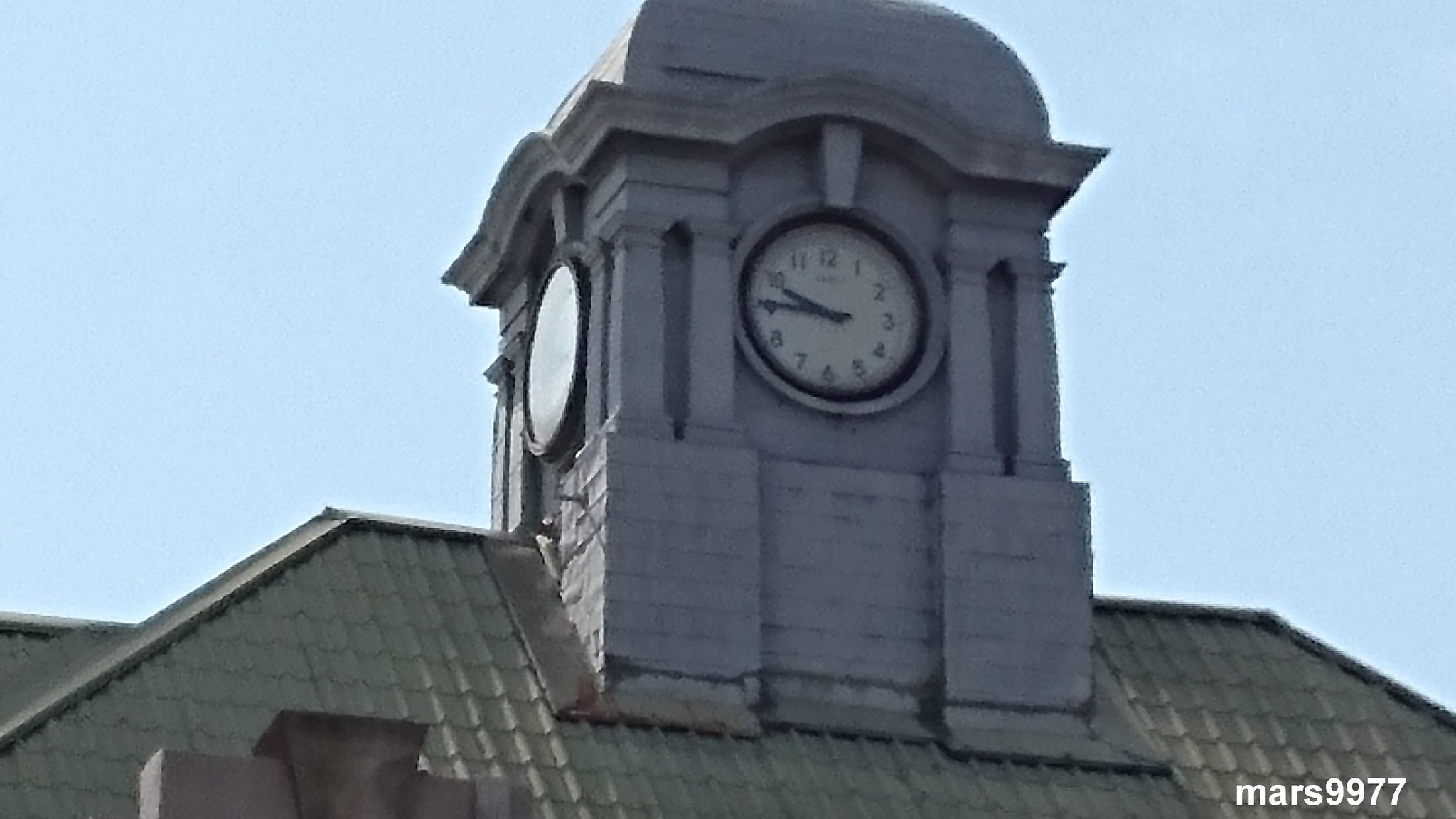This is a detailed photo taken outdoors of an older brick clock tower perched on top of a hip-style, greenish-gray tile roof. The clock tower features intricate stone columns flanking the clock faces and has clocks on all four sides, although only two are visible in this specific shot. Each clock displays the time as 9:45, and the clock faces are designed in a classic black and white style with regular numerals. The roof of the clock tower itself is dome-shaped and made of concrete. The background includes a chimney and the sky appears to be blue, suggesting it is likely morning. The words "Mars 9977" are visible, possibly indicating the brand of the clock or the photographer's watermark.